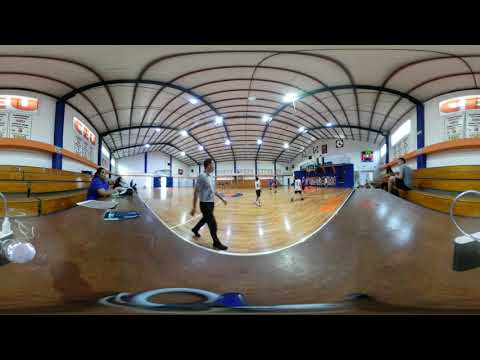The image is a low-resolution panoramic photograph of an indoor gymnasium, taken with what appears to be a 360-degree camera, causing some warping especially around the edges and a distortion of proportions. The gym features a light blonde wooden parquet floor that forms a basketball or sports court. The ceiling is notably high and predominantly white, supported by dark blue metal beams that crisscross in curved patterns. Along the left and right sides of the gym, there are wooden bleachers where some people are seated. The walls of the gym are white, adorned with various banners and signs, including prominent ones with the bold orange letters "C E U". In the foreground, a dark wooden table stretches across the image, with a person in a blue shirt leaning against it. Just left of the center, a man with dark hair, wearing a white shirt and black pants, can be seen walking across the court. In the distance, some players in white jerseys are visible, although details are hard to discern due to the image's low resolution and curvature. The image is framed by thick black rectangles at the top and bottom, further emphasizing its wide, rectangular shape.